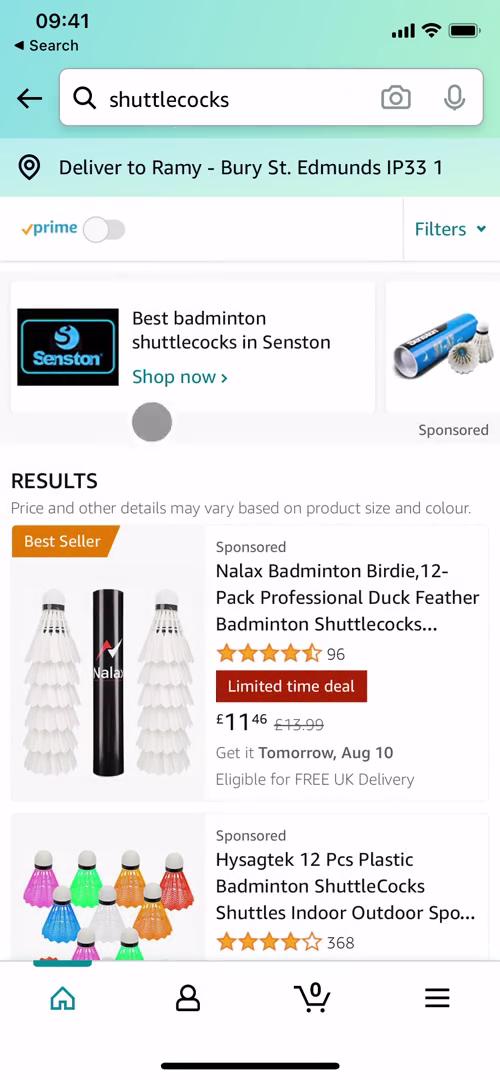The image is a detailed screenshot of a website displaying badminton shuttlecocks. The top of the screen has a gradient background transitioning from turquoise to a sea glass green color. The time "09:41" is displayed at the top-left corner, with icons for battery, cell signal, and Wi-Fi signal on the top-right.

Below the time is a grey navigation bar featuring a left-pointing arrow, a search bar with the word "shuttlecocks" written in it, a black magnifying glass icon, a camera icon, and a microphone icon. The search bar itself has a white background.

Underneath the navigation bar, the background transitions to a lighter blue hue blending into sea green. It displays the current delivery location as "Delivery to: Ramy, Bury Street, Edmonds, IP33 1". A "Prime" indicator suggests the Prime service is turned off. There are filter options presented in teal text along with a dropdown menu.

The search results section begins with a header indicating "Best Match: Best Badminton Shuttlecocks by Senston", followed by a "Shop Now" button and a "Sponsored" label. Additional text underlines that prices and details may vary based on product size and color. 

The first product listed is tagged as "Bestseller" and "Sponsored", describing "Nalax Badminton Birdie, 12-pack Professional Duck Feather Shuttlecocks" available for a limited-time deal at £11.46. The following item, also labelled "Sponsored," showcases "Hike Cyc Tech, 12-piece Plastic Badminton Shuttlecock Shuttles, Indoor Outdoor Sports."

The comprehensive display provides users with detailed options and filters to refine their search for badminton shuttlecocks.